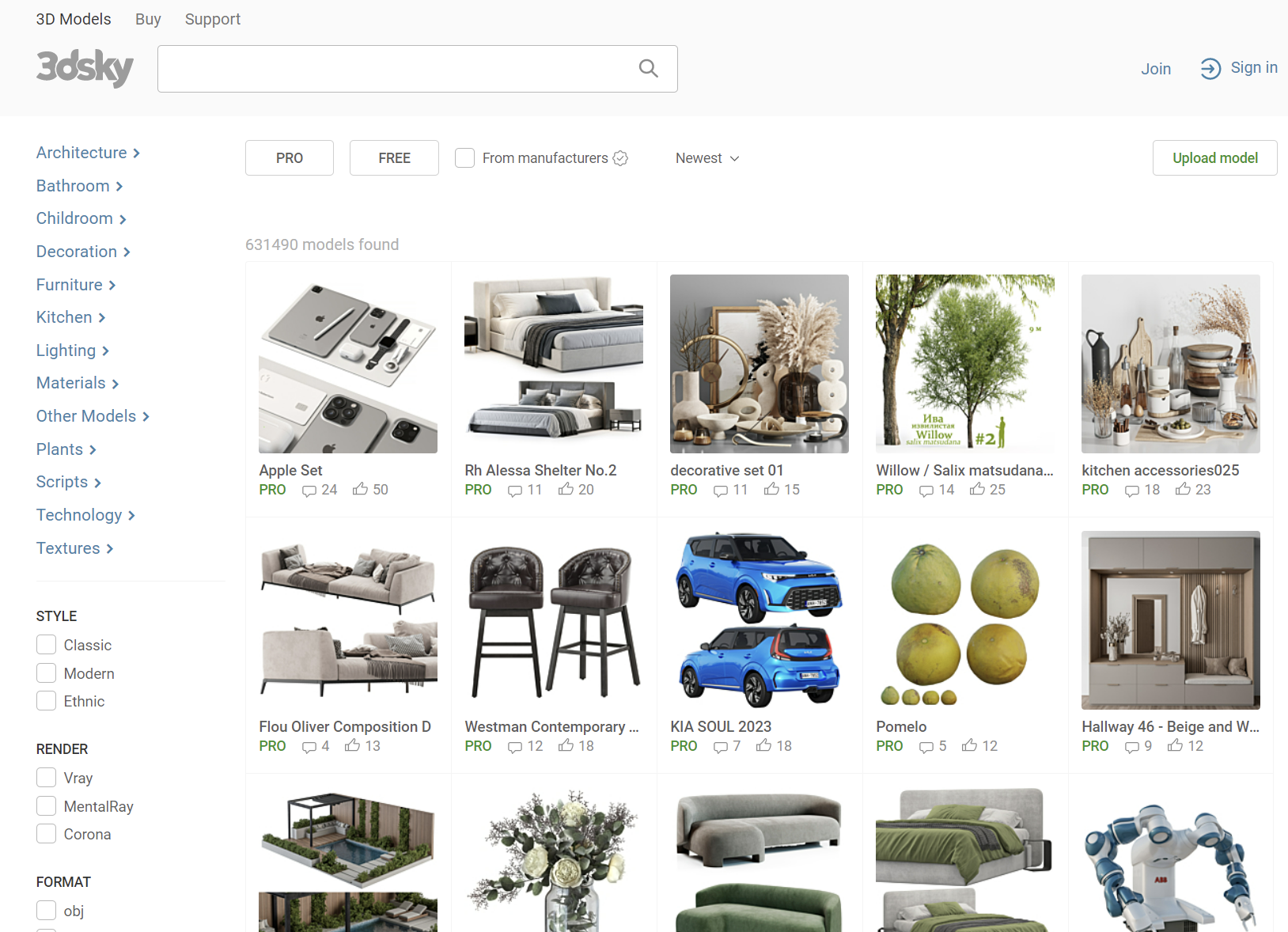This image captures the homepage of the 3DSKY website, a platform for purchasing 3D models. At the top of the page, there is a faint gray rectangle banner featuring navigation options. On the left, the site's name "3DSKY" is prominent, followed by a search bar with a gray magnifying glass icon. Adjacent to the search bar, "3D Models," "Buy," and "Support" options are displayed. To the right, there are links to "Join" and "Sign In."

Below the top banner, the navigation sidebar on the left lists various categories such as Architecture, Bedroom, Children, Decoration, Furniture, Kitchen, Lighting, Materials, Other Models, Plants, Script, Technology, and additional filter options for Style, Render, or Format.

The main content area showcases a variety of available 3D models for purchase. Some highlighted models include the "Apple Set," "Alicia Shelter No. 2" (which appears to be a bed), a "Decorative Set," "Willow Salix" (resembling a tree), "Kitchen Accessories," and a "Kia Soul." Other featured models include "Pomelo," "Westman Contemporary," and an assortment of other intricate and diverse 3D models catering to different needs and preferences.